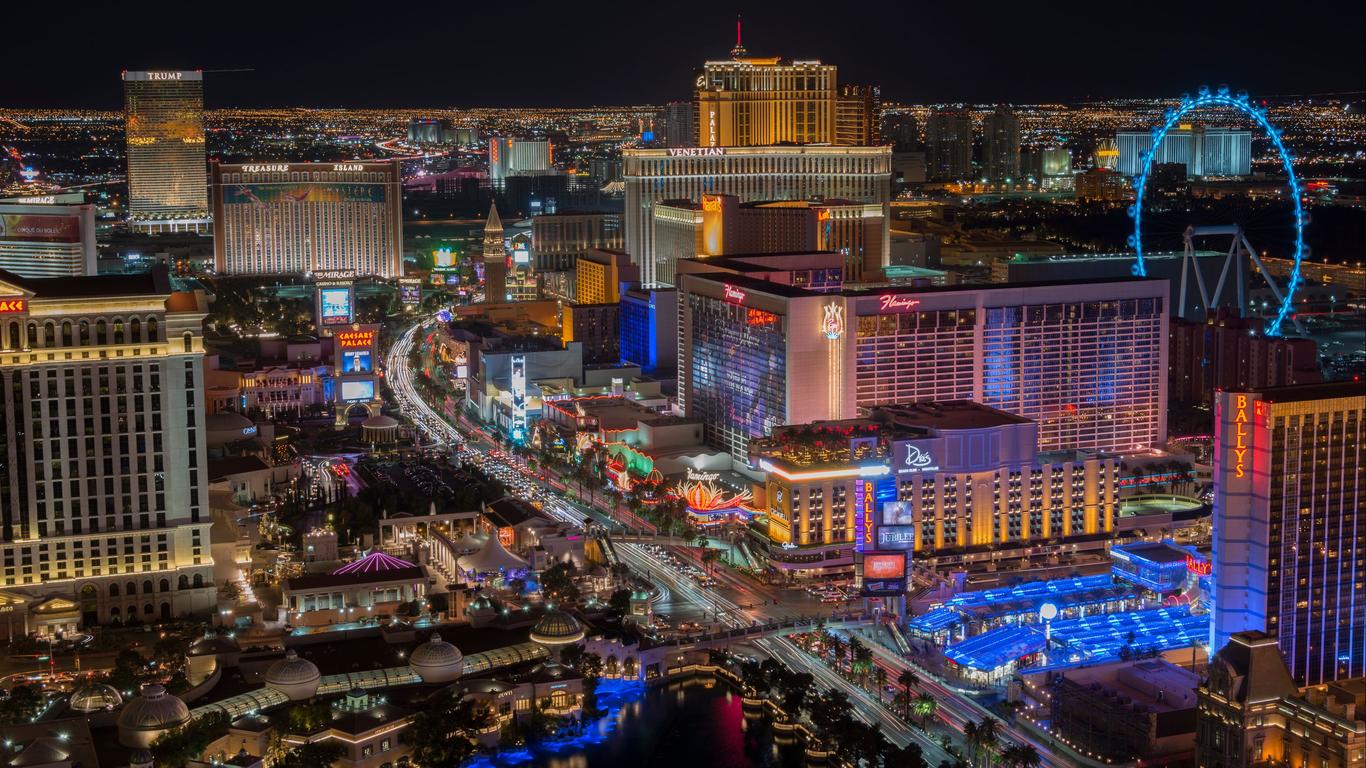This photograph captures an expansive cityscape at night, taken from a high vantage point, possibly a tall building or an aerial perspective. The skyline is densely packed with both towering skyscrapers and shorter buildings, some illuminated in purple and yellow hues. In the center, a main road is clearly visible, dotted with numerous headlights from the vehicles below, creating a lively stream of light. To the right, a large circular ferris wheel, glowing blue, adds a whimsical element to the urban scene. The city stretches infinitely towards the horizon, the lights blending into the night, beneath a pitch-black sky.